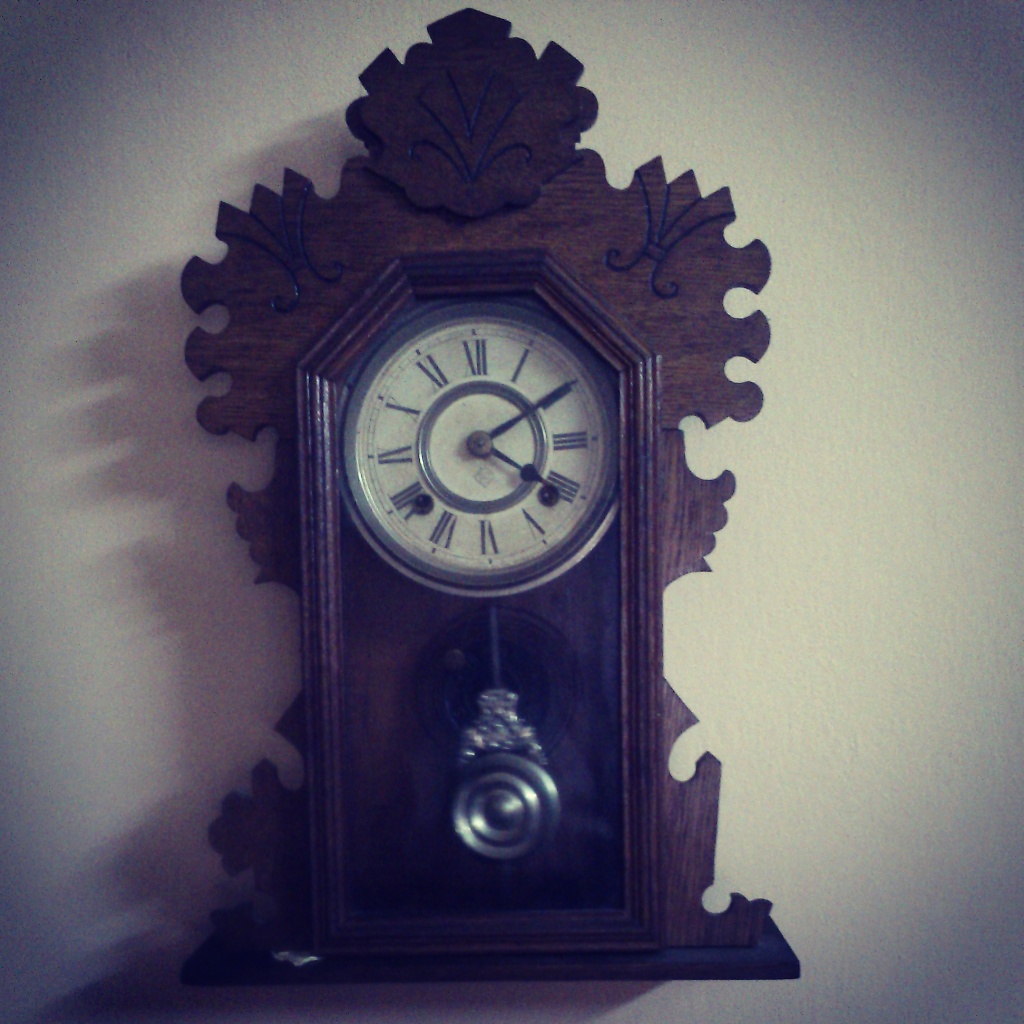The image features a rather unique and decorative wooden clock set against a gray background that fades to darker shades towards the corners. The central focus of the image is the clock, which hangs on the wall, creating a shadow to its left. This clock boasts an intricate design with irregular-shaped carvings on both sides, resembling a jigsaw puzzle. Its standout feature is the six-sided wooden frame that encases a round white clock face with Roman numerals, bordered by a shape reminiscent of a coffin. The clock's arms are set at 4:10, and a silver pendulum hangs from the bottom. The overall craftsmanship of the clock is quite detailed, featuring dark brown wood with visible lines and professional carvings, augmented by some decorative black elements that enhance its aesthetic appeal. The pendulum and other metallic parts reflect light, adding a touch of elegance to its robust wooden structure.